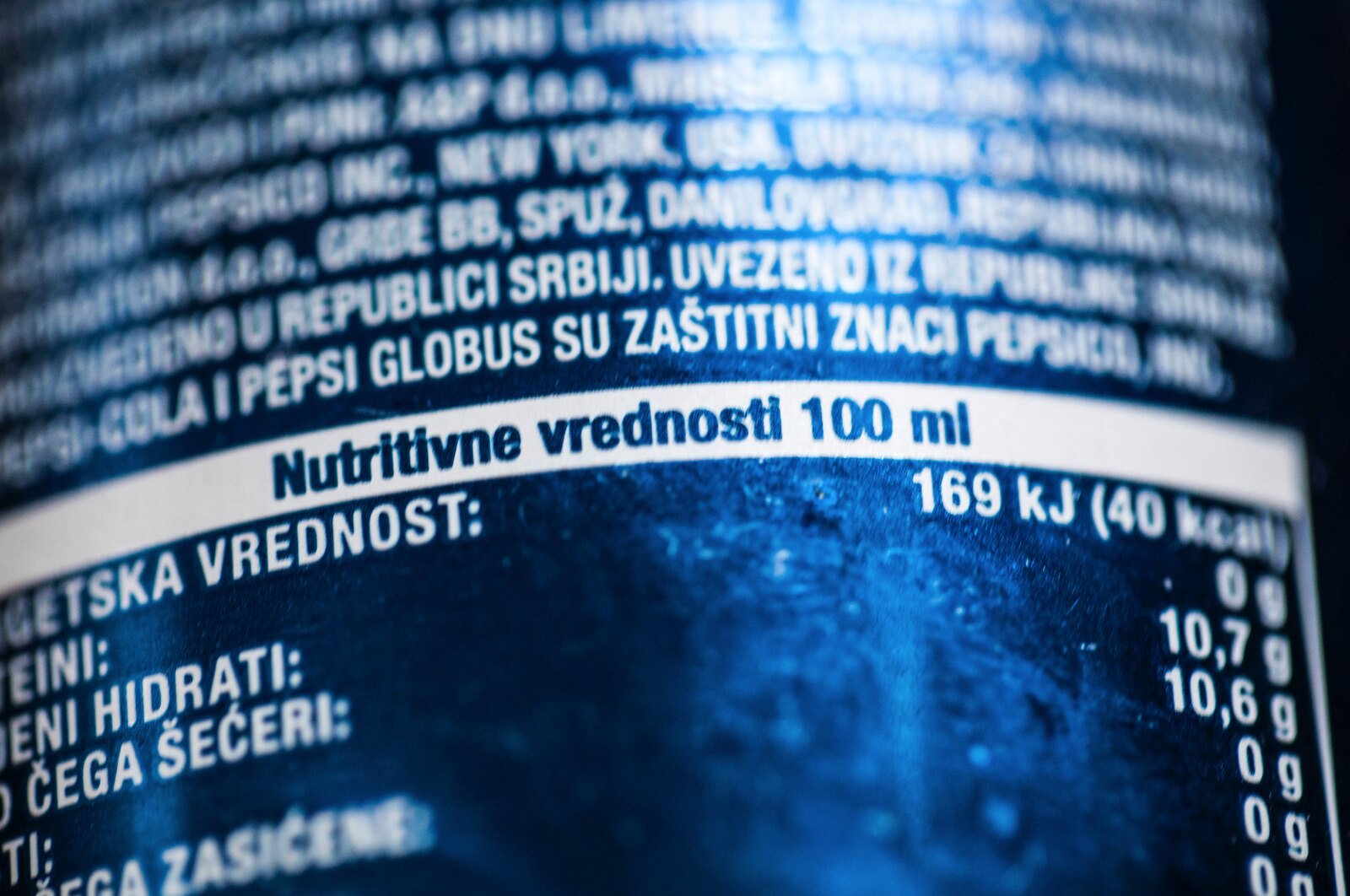This image features an extreme close-up of a dark blue, possibly sapphire to royal blue, Pepsi can from another country. The visible portion of the can is dominated by a white banner with blue text that reads "NUTRITIVNE VREDNOSTI" and lists nutritional facts for 100 milliliters. The text is in a different language, possibly Russian or Eastern European, with details such as "169 kilojoules" and "48 kcal" clearly visible. Above the nutritional facts are ingredients and addresses, featuring the term "New York, USA" amid the foreign text. The lower part of the visible section includes various nutritional values in a language that is not easily decipherable, but recognizable English words like "Pepsi" and "Cola" suggest it may be a sugar-free version of the drink.